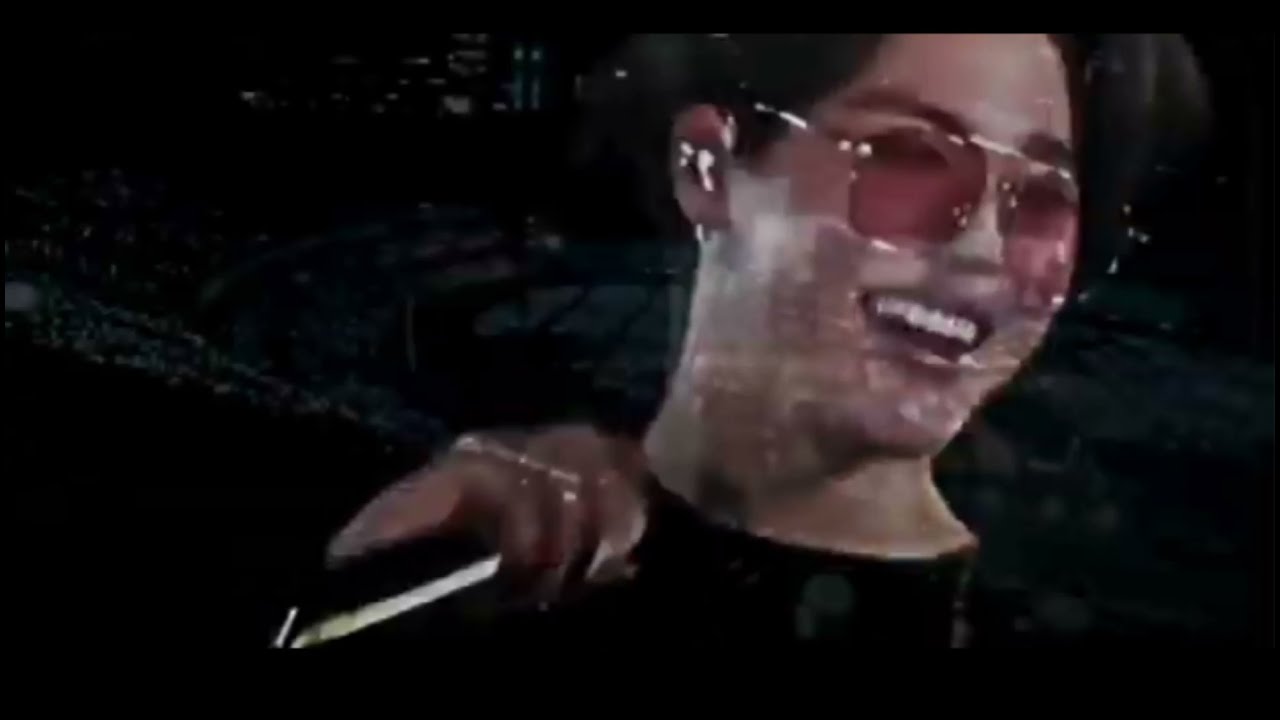In this wide rectangular image of a likely concert scene, an Asian young man takes center stage against a predominantly dark, blurry, and ambiguous background that may resemble a concert arena. He is captured from the chest up, smiling brightly with his top white teeth visible, and is facing toward the right. His expressive face is highlighted by bright pink, rose-tinted glasses, and he holds a microphone close to his neck. The young man’s short black hair and black t-shirt stand out in the focused lighting. His image appears somewhat transparent, allowing the indistinct background to subtly show through, adding an ethereal quality to the photograph or digital artwork.